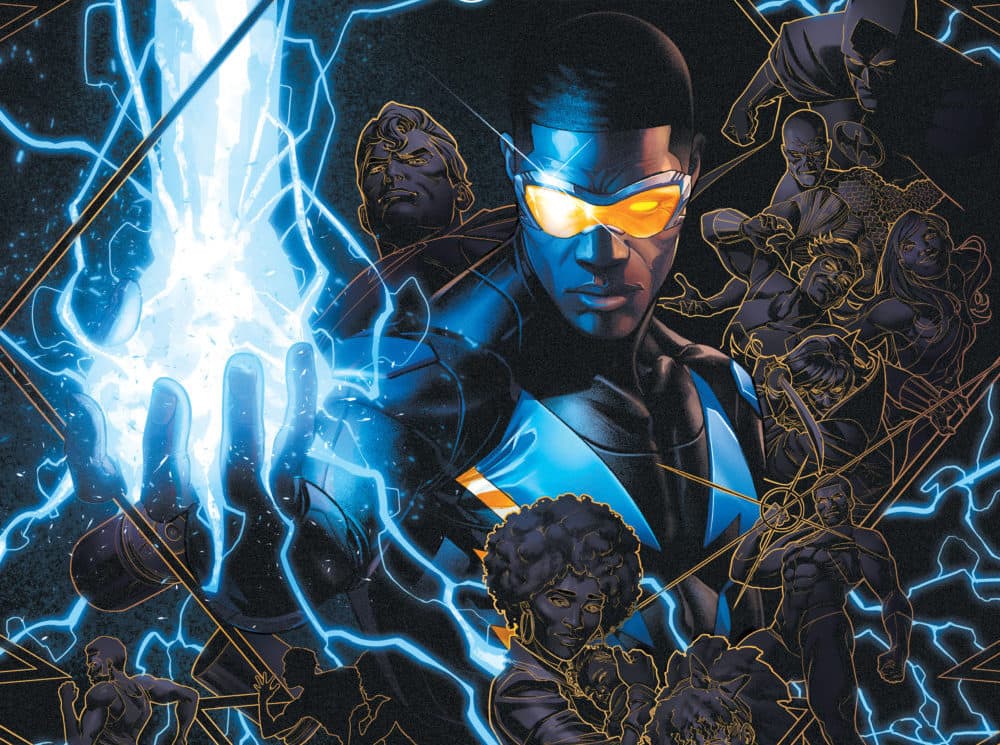This highly stylized comic book image prominently features an African-American superhero wearing yellow goggles, a blue, black, and golden costume. He extends his hand towards the viewer, emitting powerful lightning or energy. Rendered in a striking 3D effect, the main character commands attention. Surrounding him are various smaller, more subtly depicted figures in black with golden outlines, creating a dynamic relief pattern. These figures include diverse characters such as a mother holding a baby, a bodybuilding man, and iconic figures like Superman looking down. The composition suggests a mix of heroes and villains, adding depth and intrigue to the scene.